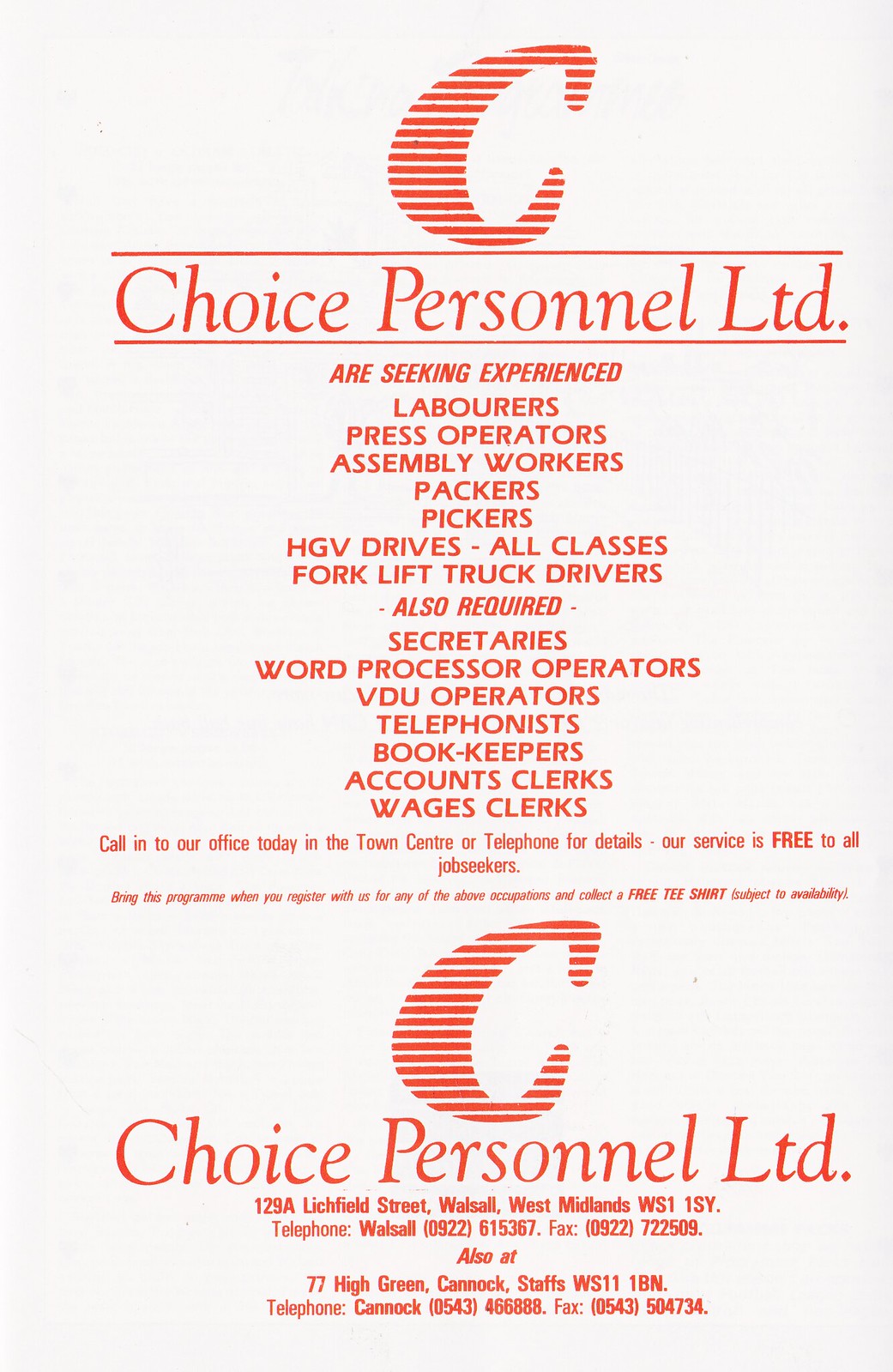This color photograph showcases a vintage advertisement on an off-white background with bright red-orange text. Dominating the top of the ad is a prominent, stylized letter "C" composed of horizontal lines. Below this graphic, centered on the page, the heading reads "Choice Personnel LTD" in bold red font. 

The ad seeks experienced laborers, press operators, assembly workers, packers, pickers, HGV drivers (all classes), forklift truck operators, secretaries, word processor operators, VDU operators, telephonists, bookkeepers, accountants, clerks, and wages clerks. Potential applicants are encouraged to visit the office located in the town center or call for further details. It is emphasized that Choice Personnel LTD offers a free service to all job seekers. Additionally, those who bring in the advertisement when registering are eligible to receive a free t-shirt, subject to availability.

The ad also includes the company's complete address and contact details: 
129A Litchfield Street, Walsall, West Midlands, WS1 1SY, Telephone: Walsall 0922. There's a secondary office address at 77 High Green, Cannock, Staffs, WS11 1BN.